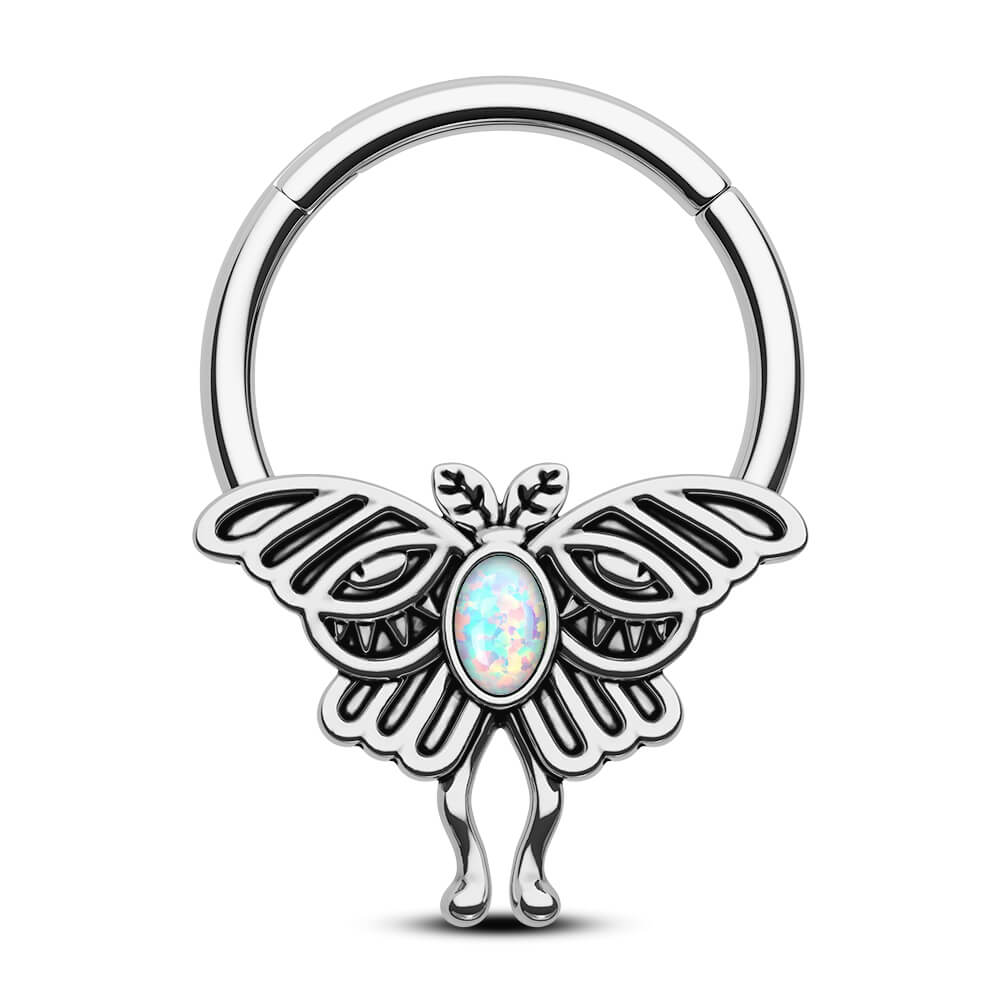The image features a brightly polished silver ring resembling a butterfly. The ring is displayed with its typically top part resting on the bottom, highlighting its unique design. The butterfly motif is detailed with wings, two legs at the bottom, and delicate feelers. At the center of the butterfly lies an oval, egg-shaped opal stone that shimmers with multicolored hues of greens, pinks, and purples. The ring's band includes two slits, suggesting it could also function as a versatile keychain. The legs of the butterfly appear to hold the entire structure, giving the piece a distinctive and elegant appearance.